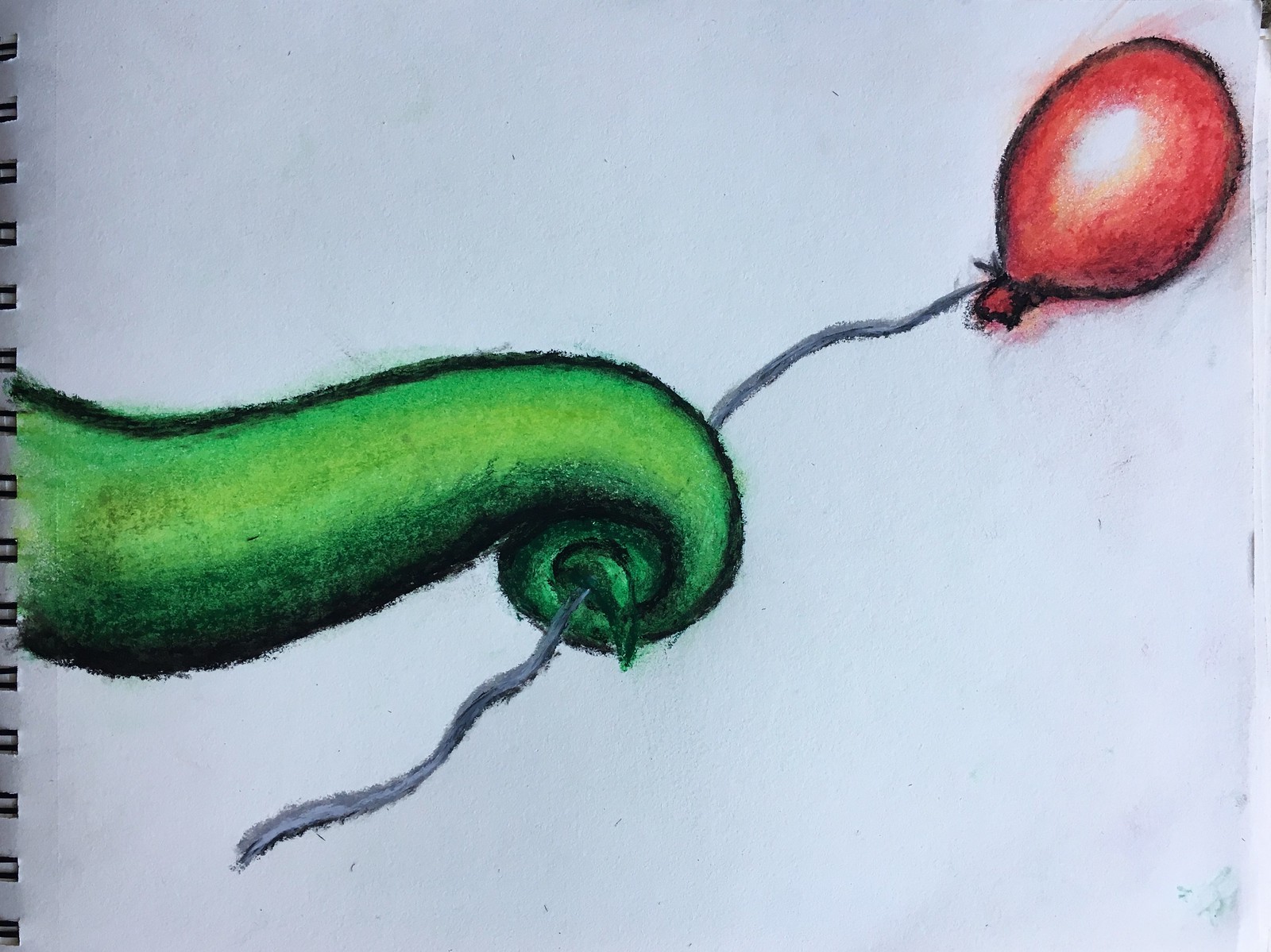In this detailed drawing on a white spiraled sketch pad, the artist has used a technique resembling pastels, chalk, or crayons. The central figure in the artwork is a vivid green tentacle, potentially the arm of a mythological creature or an octopus. The tentacle, which also features subtle hints of yellow to enhance its depth and realism, winds through the page from the left. Its sinuous form is carefully outlined in black, accentuating its twists and turns. Entwined within the tentacle is a black-gray string attached to a red balloon, which appears to float diagonally towards the top right corner of the image. The balloon, outlined in black and colored in with a glossy red hue, catches the viewer's eye with a highlighted spot that gives it a three-dimensional, shiny effect. Evidence of the artist's physical engagement with the page is visible through smudge marks at the bottom, adding a tangible and organic feel to the illustration.